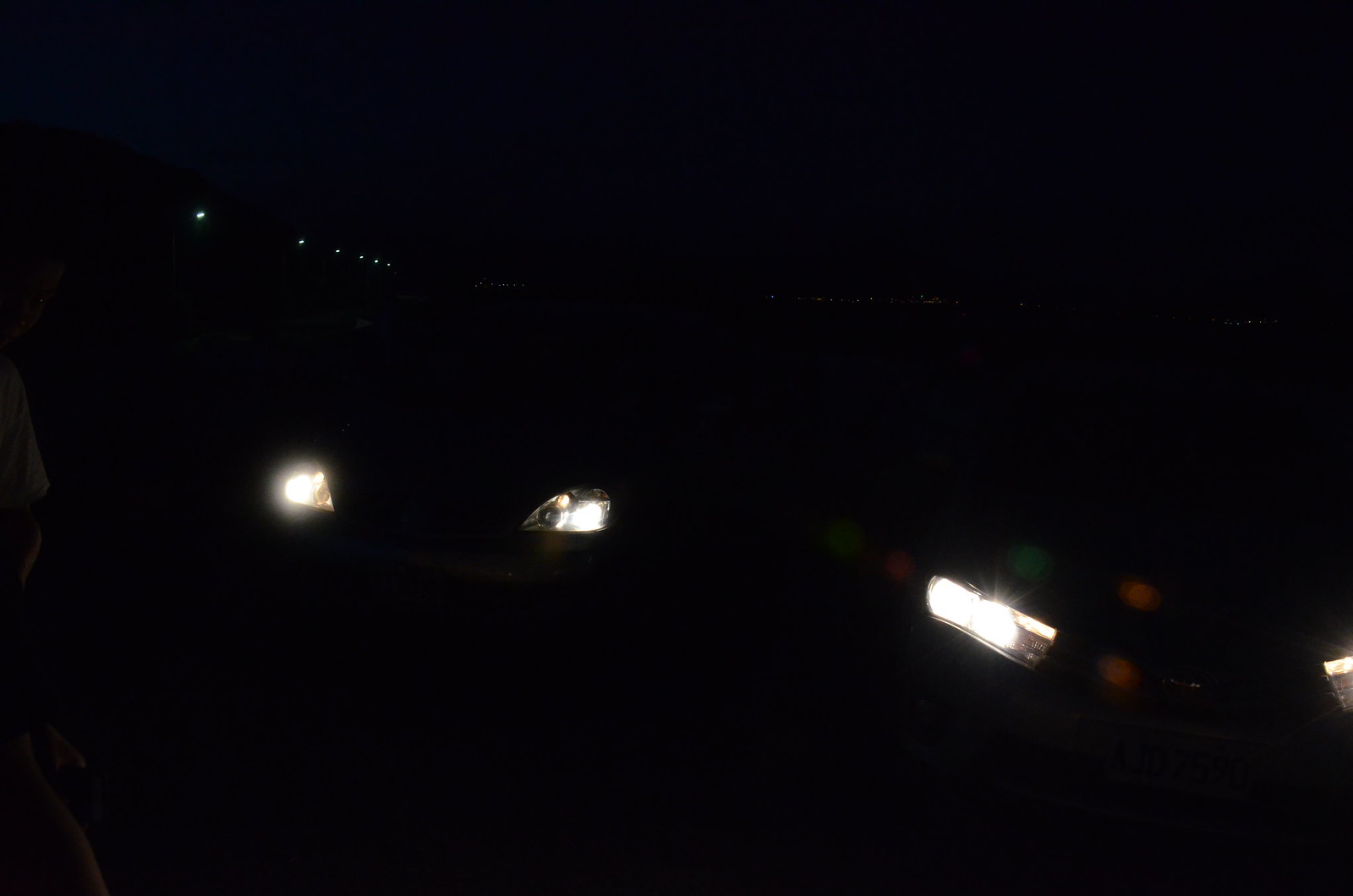This photograph captures a dimly lit, ambiguous environment that is difficult to discern whether it is indoors or outdoors. Dominated by darkness, there are notable features visible. In the foreground, multiple vehicle headlights pierce through the blackness. On the lower right, there's a visible part of a rectangular-shaped headlight, while more centrally and slightly to the left, two teardrop-shaped headlights shine brightly. Another rectangular headlight is partially visible on the edge of the image. Further back in the background, a sequence of six bright white lights dots the top half of the frame, forming a diagonal pattern. These small, circular lights add depth to the scene and may suggest distant city lights. Overall, the sparse illumination from the headlights and distant lights highlights the enigmatic and somber atmosphere of the image.